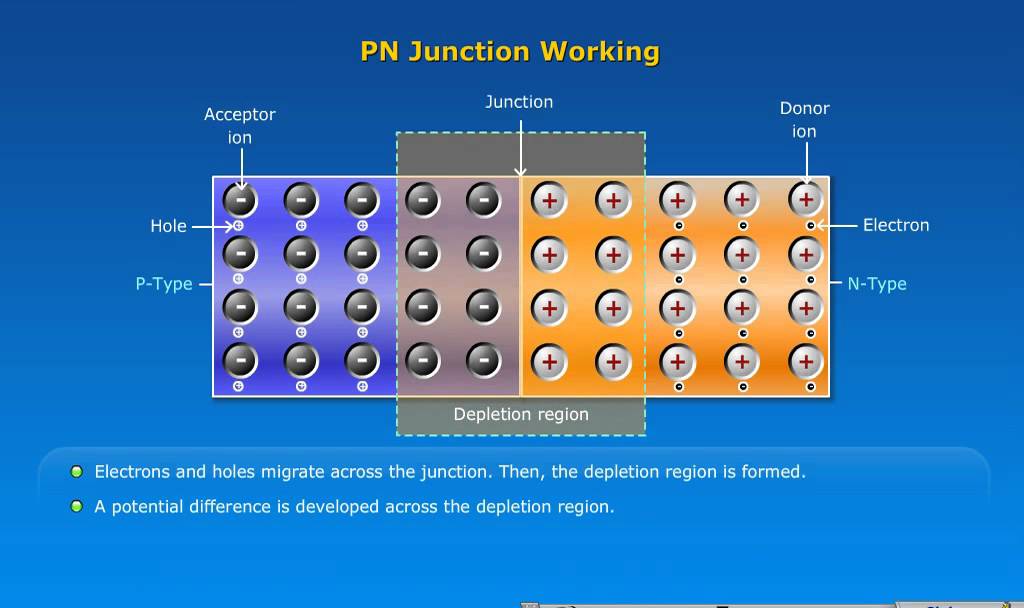The image is a detailed scientific diagram illustrating the working of a P-N junction. The background transitions from a lighter to a darker blue as it ascends. At the top of the diagram, the title "P-N JUNCTION WORKING" is prominently displayed in yellow, all-capital letters.

The diagram itself is divided into four sections. The left side features a blue background with 12 circles, each containing a minus sign, accompanied by labels: "Acceptor Ion," "Hole," and "P-Type," with arrows indicating their positions. The central section is a pinkish-purple color marked as the "Junction," and the right side is orange, segmented into two parts, each filled with circles bearing plus signs. The labels in the orange sections include: "Donor Ion," "Electron," and "N-Type."

Surrounding the central junction area is a spotted light blue line with a gray border, indicating a boundary. Below the sections, there is a label "Depletion Region." At the very bottom of the diagram, explanatory text reads: "Electrons and holes migrate across the junction. Then the depletion region is formed. A potential difference is developed across the depletion region."

The diagram visually and textually captures how charge carriers (electrons and holes) migrate across the P-N junction, resulting in the formation of a depletion region and a potential difference.